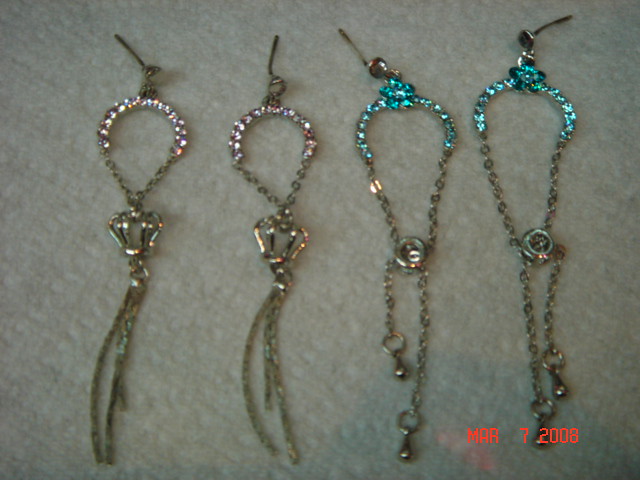A detailed photograph from March 7th, 2008, captures two pairs of intricately designed, large dangly earrings displayed on a white cloth surface, with the date marked in pixelated red font at the bottom right. The earrings are arranged side-by-side in the image, viewed from above.

The pair on the left features elaborate designs with an upside-down teardrop-shaped top section adorned in pink lavender gemstones. These tops connect to chain-like structures forming a crown, from which three tassel chains hang. The earrings have bronze-colored clasps, though the right one appears slightly bent.

The pair on the right, while similar in length and style, showcases aqua blue gemstones at the top, shaped like a circular piece of metal without a crown. Instead, they have a single rhinestone flower at the center and two chain tassels ending in teardrop-shaped metal tips. 

Both pairs exude elegance, with their intricate detailing and play of colored gemstones, reflecting light and adding a touch of sophistication to the white cloth background.